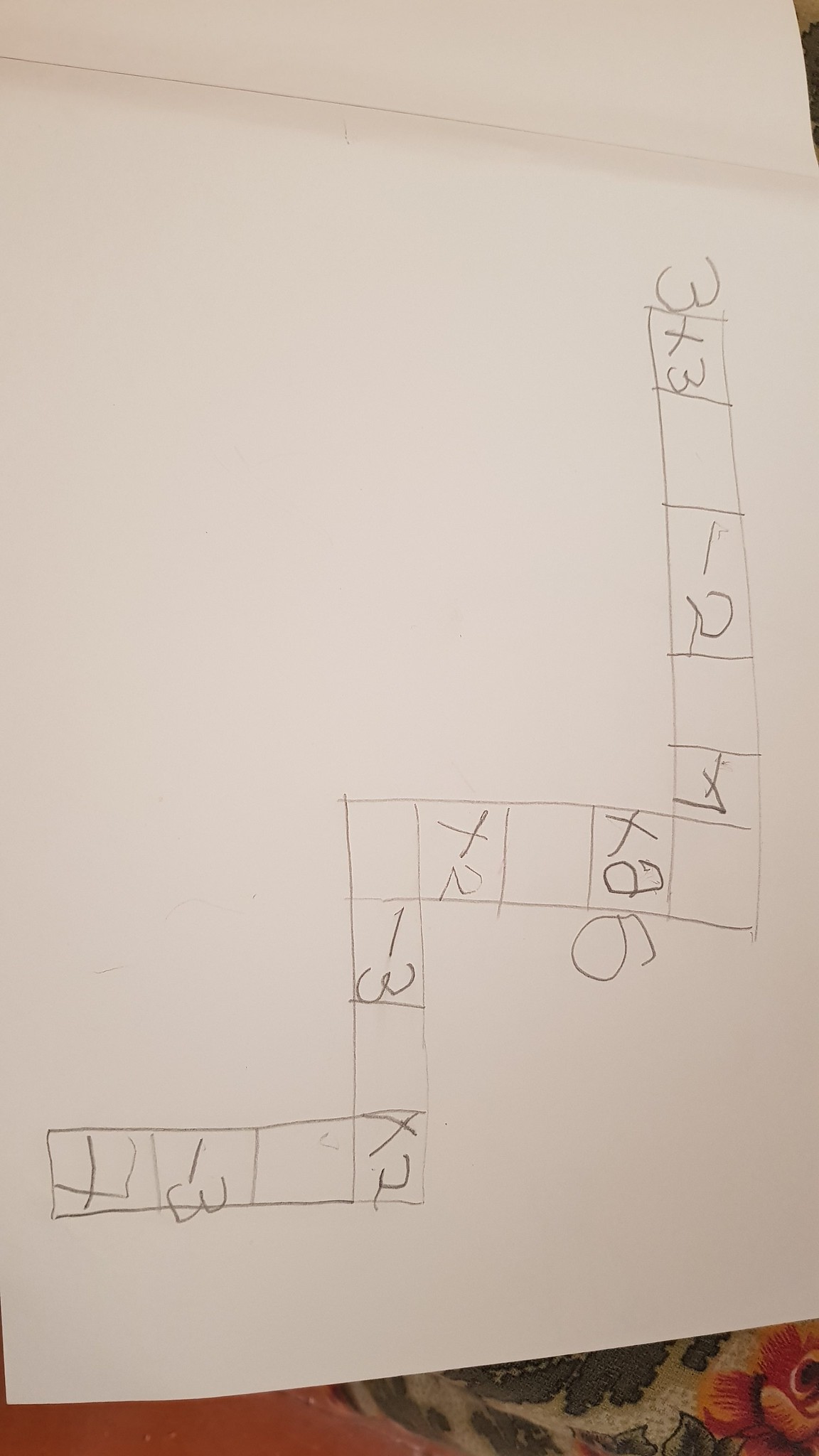The image depicts a math problem meticulously sketched on a piece of paper from a spiral-bound notebook. The notebook appears to be slightly tilted to the right, with another sheet partially visible and connected by the binding at the top, suggesting that the pages could easily be torn out when finished. The math equation is artistically represented within a series of interconnected squares. There is one vertical row of squares, which is then joined by a horizontal row. This pattern repeats, creating a formation that somewhat resembles the letter ‘Z’ with an extended tail pointing downward, giving the overall layout a distinctive and geometrically precise appearance.